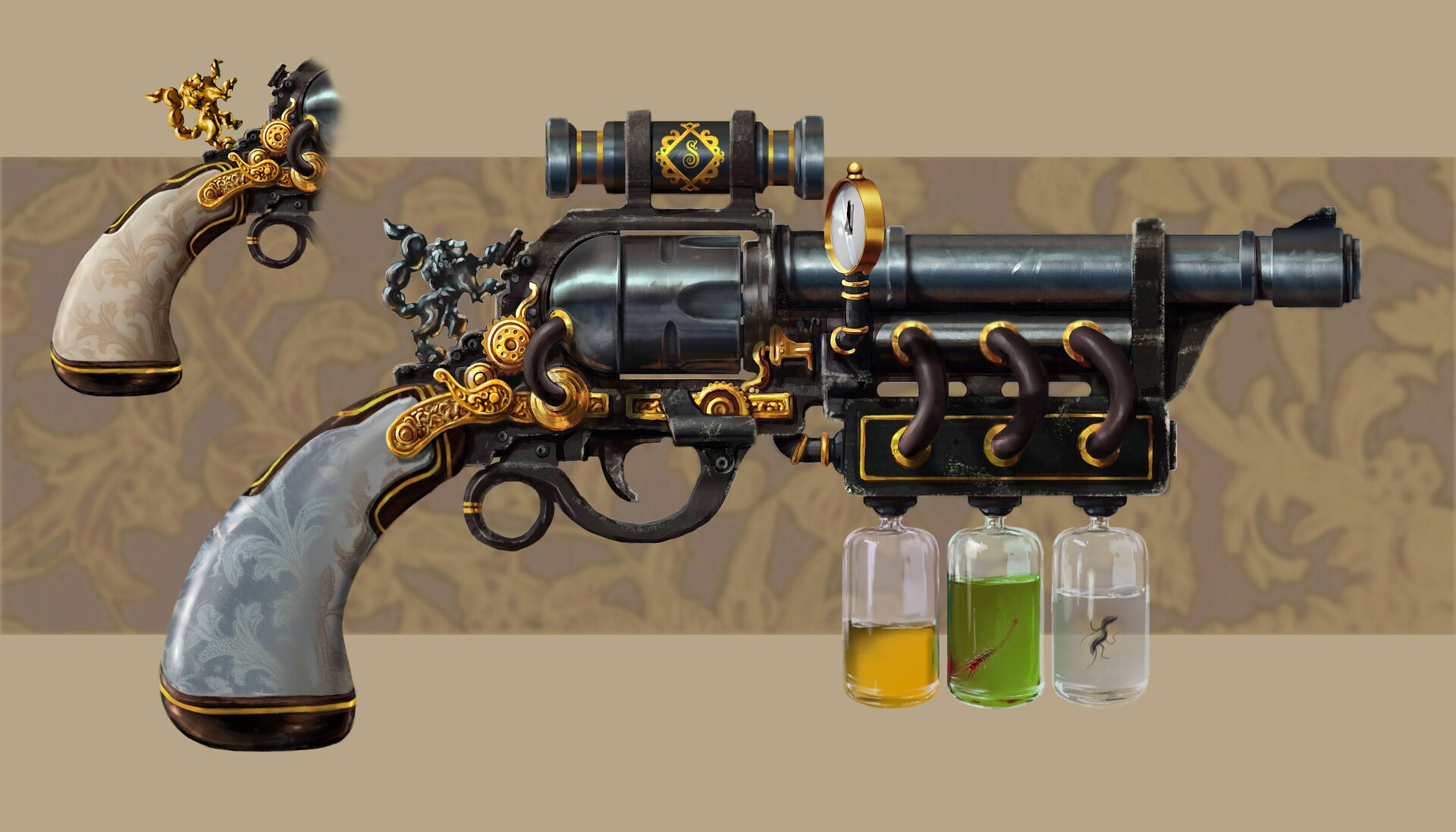This horizontal, color illustration features an intricately designed, fanciful gun prominently centered against a subtle floral cream background. The gun has an elaborate mix of materials including a matte black trigger, ornate gold adornments, and black tubing. The handle appears to be metallic with etching, predominantly black and white or gray, while another handle in the image is a darker color, suggesting a choice between the two.

A standout feature is the attachment of three glass vials beneath the barrel, each containing different colored liquids: one yellow, one green, and one clear with what appears to be a large ant inside. The gun is further embellished with flourishes, filigree, and a timer-like component, enhancing its whimsical and surreal appearance. The overall design, complemented by a telescope-like sight reminiscent of a pirate's scope, gives the impression of a fantastical creation rather than a real firearm, possibly an AI-generated or artist-imagined concept.